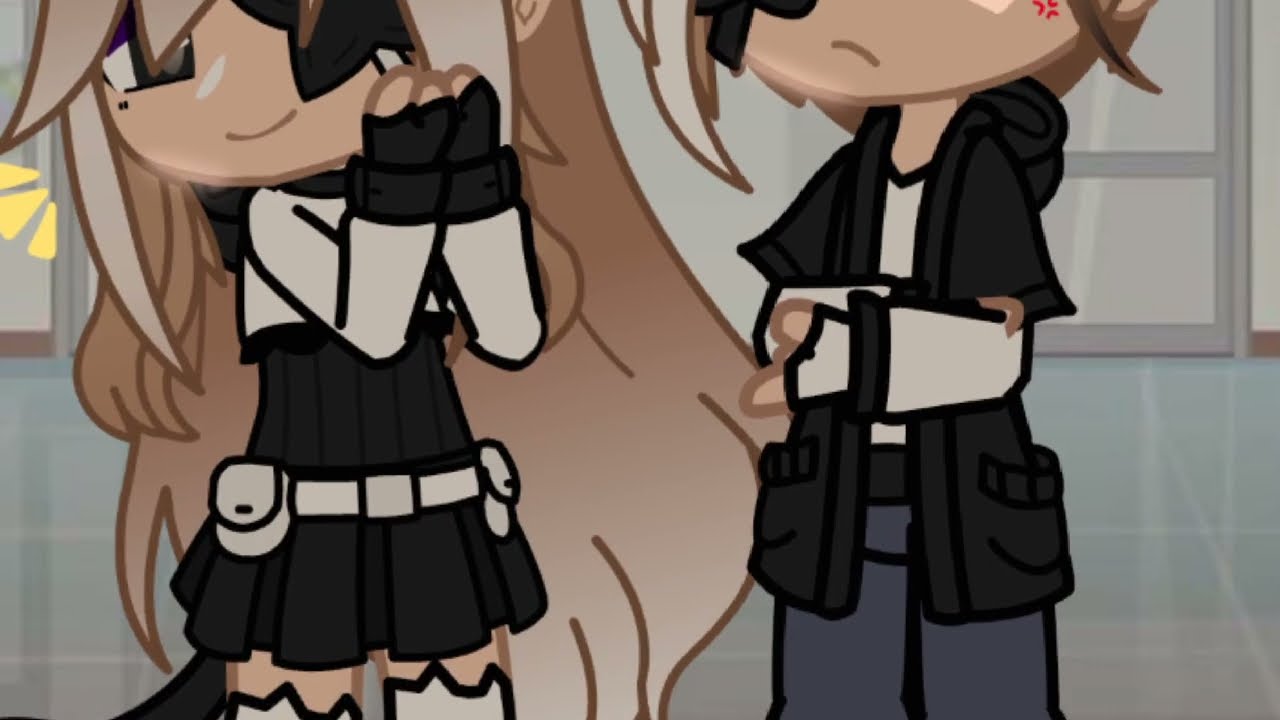A detailed cartoon drawing shows two characters against a light bluish-grey wall with a grey-framed window behind them. On the left side, a girl with long, flowing brown hair, styled with wispy pointed tips, is dressed in a white long-sleeve top under a black dress with a distinctive white belt featuring side pockets. The dress stops short, revealing a bit of her thighs above white boots. She is holding her arms up to her mouth, with her fingers sticking out from what appear to be fingerless gloves. The girl's expression hints at curiosity or amusement as she directs her gaze at the boy on the right.

The boy, standing next to the girl, wears a black coat over a white shirt with grey and brown pants. His posture is somewhat reserved, with his hands folded around his waist area. Part of his face and that of the girl’s are lightly obscured, possibly by a hairband or some accessory. The boy's expression appears more serious compared to the girl’s. This image, potentially from a comic, TV show, or movie, captures a moment of contrast between the characters' emotions and attire.